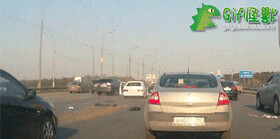A photo captures a busy highway scene with cars in motion under a clear, light blue sky. The main focus of the image is a silver sedan with its brake lights illuminated and a white, glare-obscured license plate. Surrounding this car are several others; notably, a black sedan's front end is visible in the bottom left corner, and diagonally from the silver sedan, a white car with its door open can be seen. Further ahead in the same lane as the silver sedan is a gold car. Lampposts line the road, and a small rectangular blue sign with indiscernible white lettering is on the right side. Amidst this scene, in the right-hand corner, a green dinosaur-like creature with the letters "GIF" and some Chinese characters appears, adding a whimsical touch. Signs of potential disruption are evident with the presence of debris around the silver car, hinting perhaps at a recent incident.